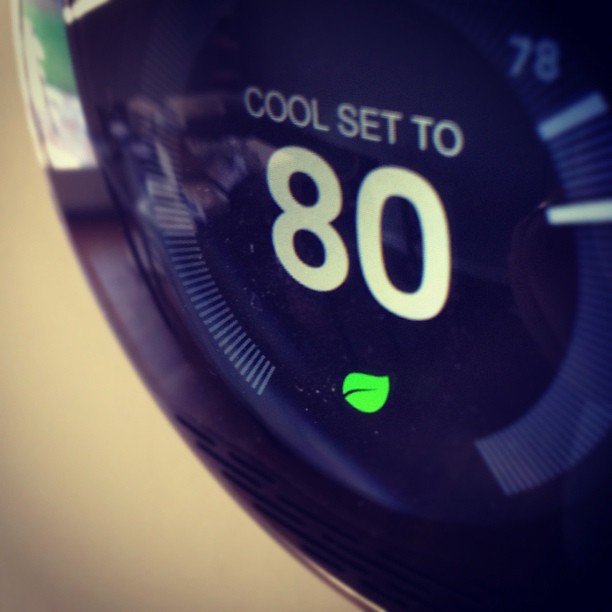The image is a close-up photograph of a digital smart thermostat, captured in a square format. The thermostat, predominantly out of frame, features only a partial view of its LED screen and the bottom left side of its casing. The photograph is taken from an angle that makes the bottom left of the thermostat appear larger than the top right, likely due to the perspective from which the photo was taken. 

The thermostat's casing is white, accented by a silver band encircling the main LED screen. The screen itself is circular and displays information in large white characters against a dark backdrop. The prominent text on the screen reads "Cool set to 80," with a small green leaf icon situated directly beneath the number 80. Additionally, the display includes two bars filled with multiple white lines on either side of the main text. On the right side of the screen, these bars feature a thick white line in the center alongside the numbers '78' presented in gray.

Overall, the photo's close-up nature and the specific angle from which it was taken emphasize the intricate details and functionality of the smart thermostat's display.